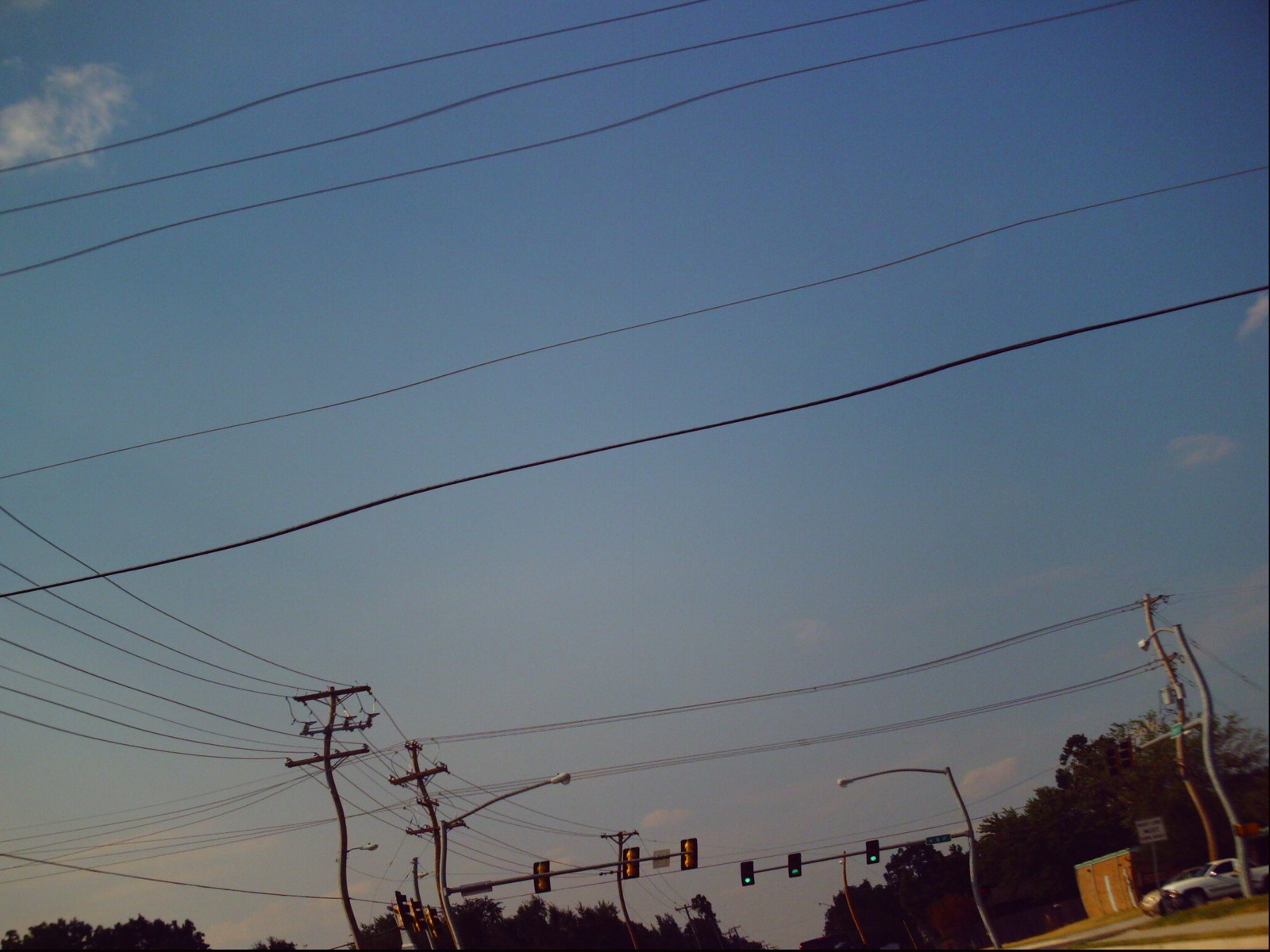The image depicts a quintessential American roadside scene captured from a low street-level perspective. Dominated by a brilliant blue sky with a few puffy clouds, the composition is replete with numerous squiggly power lines crisscrossing the view. These lines are held up by similarly distorted telephone poles, adding a peculiar, almost surreal quality to the setting. To the right, a white car navigates past a red brick station, seemingly waiting at the traffic lights which too, appear strangely wavy. The frame is ringed by towering trees, further accentuating the verticality of the power lines. Although the road itself isn’t visible, the arrangement of vertical and horizontal lines, traffic lights, and a roadway, provides a sense of an organized yet dynamic infrastructure.